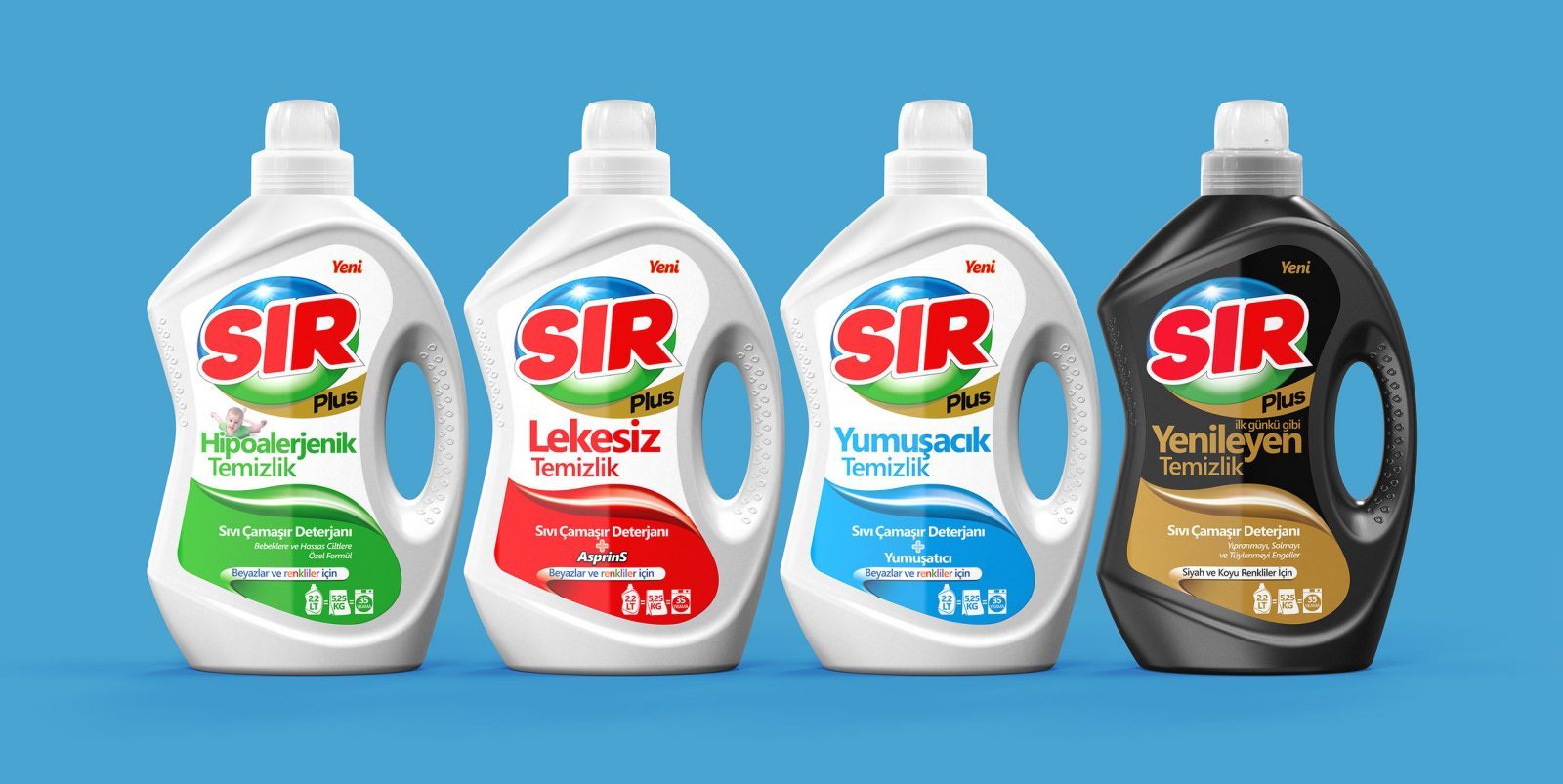The image shows four plastic bottles of laundry detergent meticulously lined up against a plain blue background. The first three bottles on the left are white, while the fourth bottle on the extreme right is black. Each bottle is adorned with a translucent white cap, and they all feature similar design elements. The bottles have handles on the right side and an indent on the left side. 

All the bottles display the brand name "Sir" prominently at the top in red text with a white outline, set against an oval logo that is blue on the top and green on the bottom, with a gold banner reading "Plus" beneath it. Additionally, each has the word "Yeni" on the upper right corner of the sticker — in red text for the first three white bottles and in gold for the black bottle. 

The text on the labels is in a language other than English, with different colored text indicating various product types at the bottom of each label. Specifically:
- The first white bottle has green text.
- The second white bottle has red text.
- The third white bottle has blue text.
- The black bottle has gold text.

Below the main logo, each bottle has specific inscriptions: 
- The first one reads "Hyperlogenic Temislic."
- The second one says "Lachesis Temislic."
- The third reads "Yumusak Temislic."
- The fourth has "Yenilean Temislic."

These bottles are arranged in a rectangular frame, approximately six inches wide by three inches high, presenting a clean, orderly appearance.